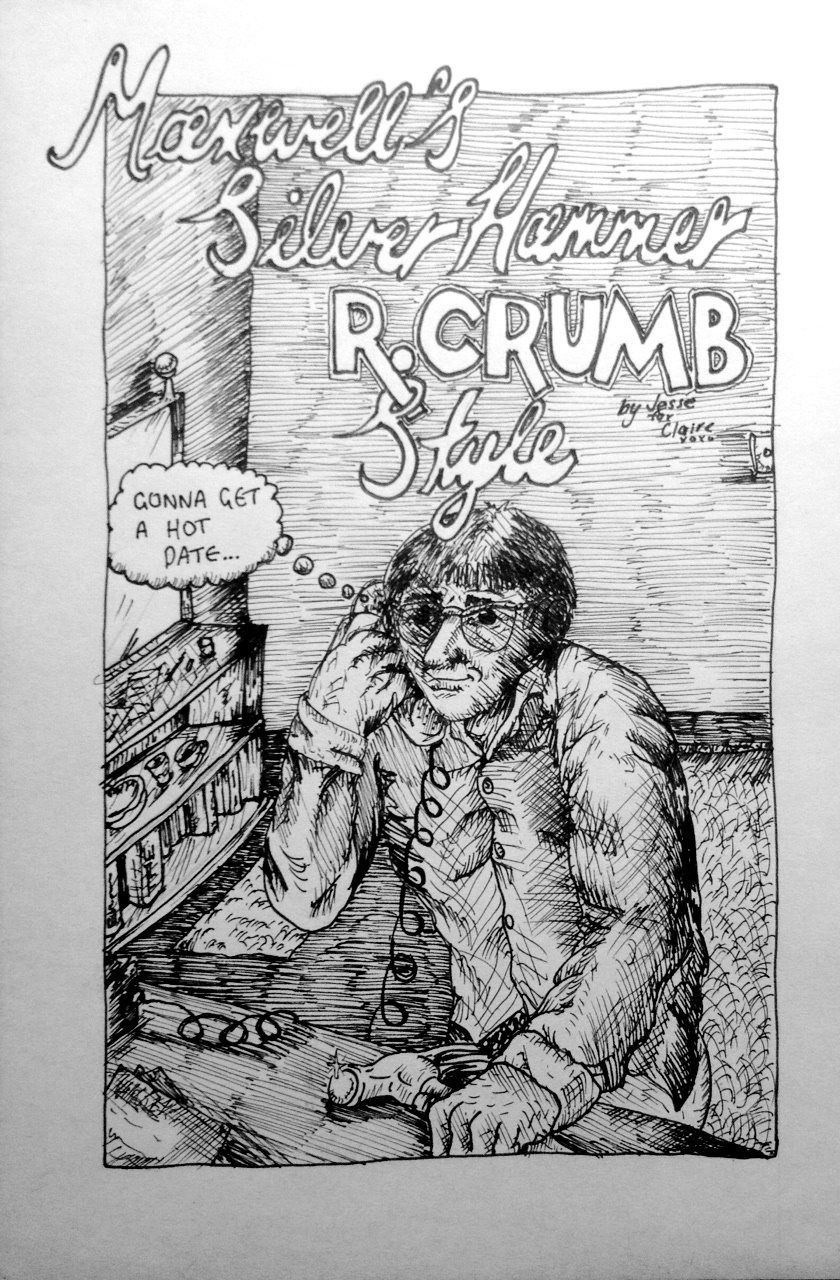The image is a detailed black-and-white line drawing styled like a comic, featuring a man with short, dark hair and glasses. At the top, the text reads "Maxwell's Silver Hammer, R. Crumb Style," followed by “by Josie for Claire xoxo.” The man, who appears to be sitting at a desk or workbench, holds a corded telephone to his right ear with a thought bubble near his head saying, "Gonna get a hot date." His left hand grasps a hammer, which rests on the tabletop. The background includes various items such as a shelf with books, cups, and plates, a TV stand or dresser, and possibly a mirror. The setting is indoors, with a carpet and a separate rug on the floor, all rendered in intricate black ink.